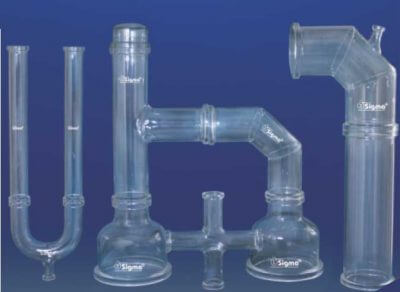The image is a wide rectangular photograph depicting an array of different transparent glass pipes and beakers set against a gradient background featuring shades of dark grayish blue, transitioning to a purple hue. On the far left, there is a prominent U-shaped glass pipe with tall sides and a smaller tube extending from the bottom where the U's sides unite. In the center, a complex glass structure shaped like a large lowercase "h" with two larger glass tubes extending out from the bottom, connected by a cross (plus sign)-shaped tube. On the right, a pipe shaped like an inverted J or candy cane extends vertically before curving to the left with a small tube protruding from the top corner. This intricate arrangement of glassware, reminiscent of a chemistry set, features numerous small tubes and openings, suggesting potential use for fluid or gas transportation. The clear glass components exhibit a light blue sheen, enhancing the detailed and scientific atmosphere captured within the luster of the vibrant background.